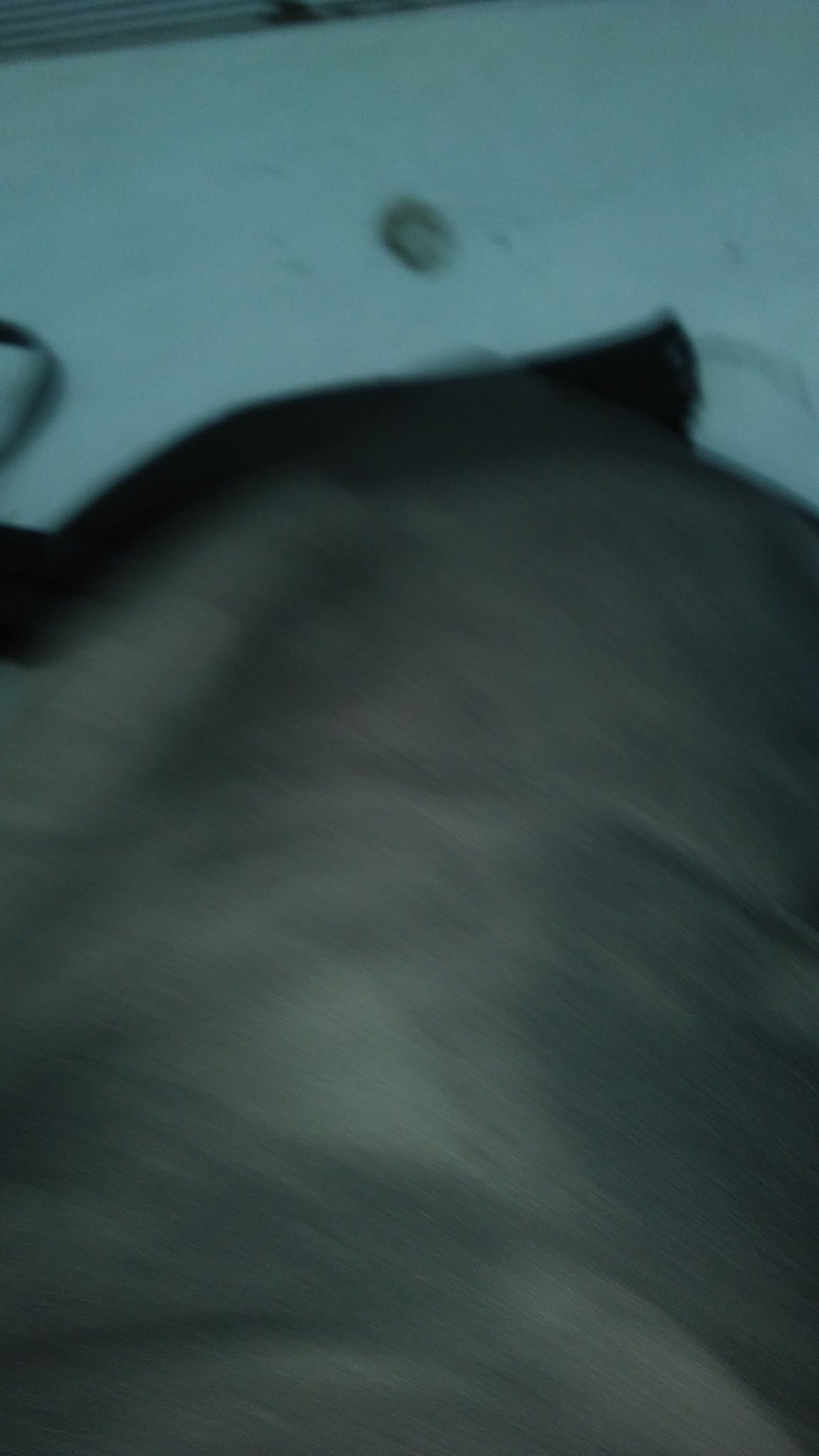This image features a rectangular frame that appears to be flipped. The overall quality is quite poor, characterized by significant blurriness and low resolution, creating a sense of motion or instability. At the top of the image, there's a prominent white area with a discernible hole in the center. Due to the blurriness, the specifics of this white section and any surrounding elements are indistinguishable. On the left side of the white area, there seems to be another object or feature, but its details are similarly lost to the fuzziness. The lower portion of the image is dominated by an expansive gray region, though its exact nature remains unclear due to the image's inherent lack of clarity.